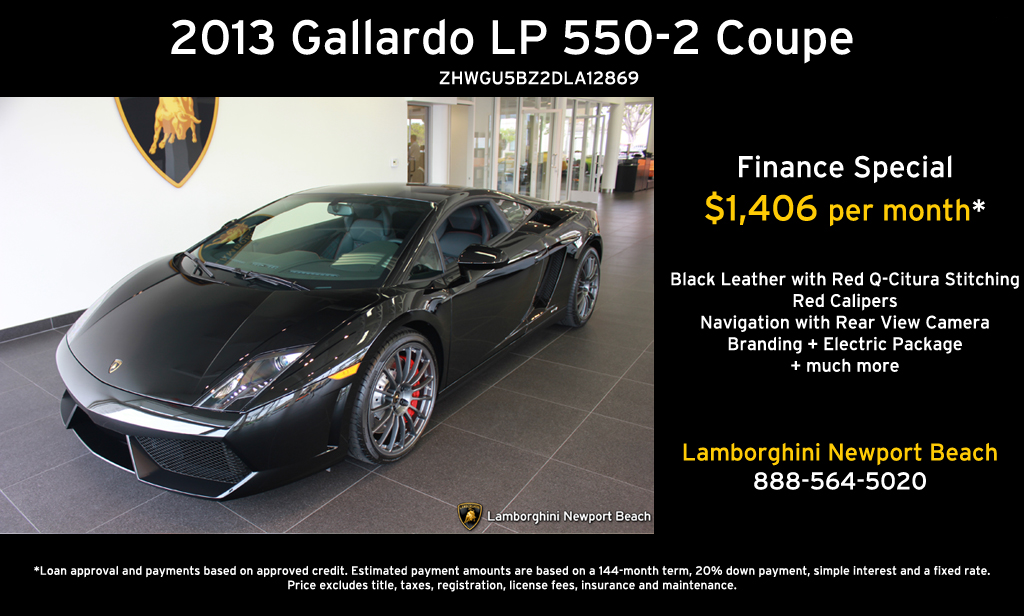This horizontal rectangular advertisement showcases a 2013 Gallardo LP 550-2 Coupe against a sleek black background. Dominating the left side is a photograph of the black car, angled to display its modern, aerodynamic design, featuring prominent wire wheels and striking headlights. The car is positioned on a floor with gray tiling, in front of a white wall adorned with what seems to be cut-off imagery, possibly an animal. Behind the car, several doors likely give entrance to a dealership showroom.

In bold white letters at the top, the ad states "2013 Gallardo LP 550-2 Coupe," followed by a line of alphanumeric code, possibly the car's serial number: "BLI 5GU 5BZ2 DLA 12869." On the right side, the ad promotes a finance special, offering the car at $1406 per month, highlighted in orange.

Additional details about the car are listed in white text, emphasizing luxurious features such as black leather seats with red "5GU-Citura" stitching, red calipers, navigation with a rearview camera, a branding and electric package, and more. The dealership's information, "Lamborghini Newport Beach," stands out in yellow, followed by the contact number "888-564-5020."

Fine print at the bottom, barely legible, mentions details about loan approval and payment conditions based on approved credit, ensuring comprehensive information for prospective buyers.